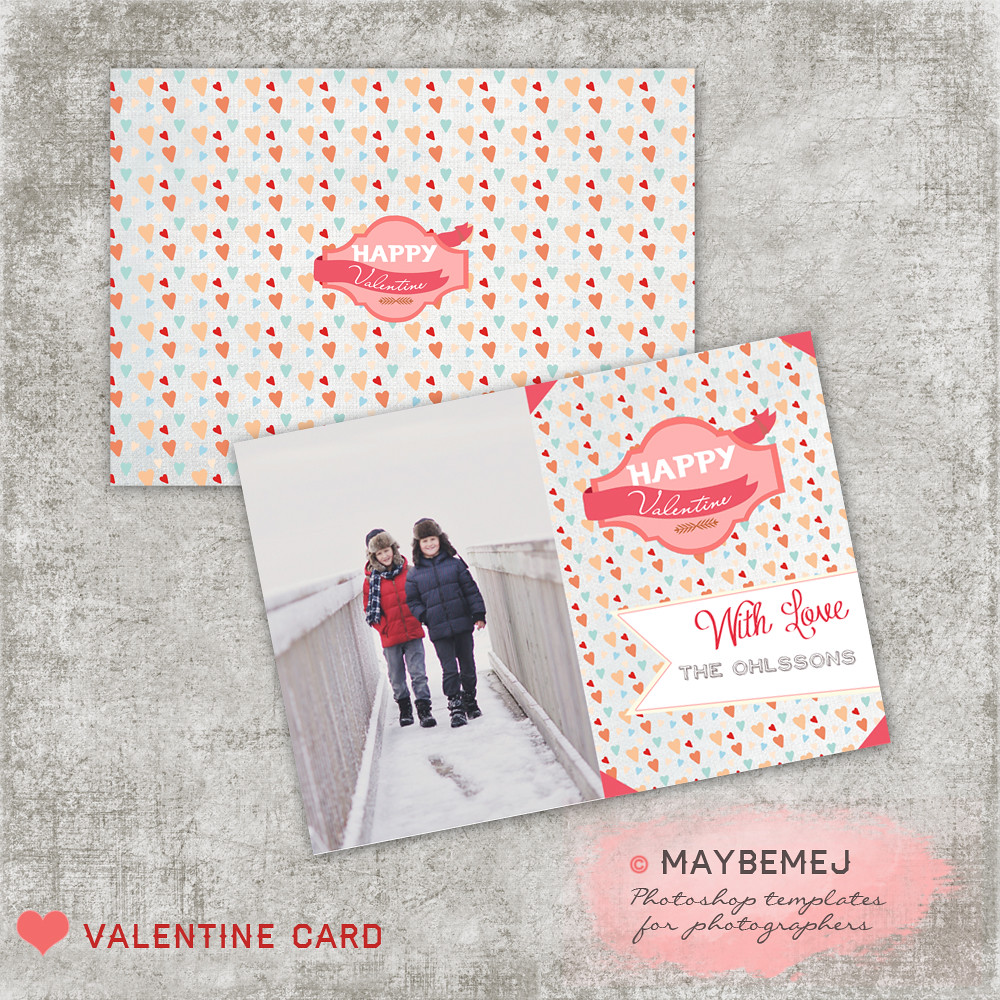The image showcases a detailed and colorful Valentine's card set against a gray and white background. One card is positioned at the top, adorned with an array of small hearts in varying colors—peach, red, pink, and light blue—scattered across a white background. In the center of this card, there is a plaque-shaped emblem with a dark pink surround. Inside the emblem, light pink and white lettering reads "Happy Valentine," with a decorative ribbon wrapped around it, its edges waving.

Below the top card, intersecting and slightly tilted to the left, is another card, or possibly a view of the reverse side of the same card. This card maintains the same heart pattern and central emblem design that reads "Happy Valentine." Additionally, there is a white banner beneath the emblem that says "With Love, the Olsens." On the left side of this arrangement, there is a photograph of two boys, approximately 10 to 11 years old, walking on a snowy dock with wooden railings on either side. Snow is visibly present on the ground and railings.

At the lower part of the card, it states "Valentine's card" in red text and possibly "beachy" in black text. A red patch at the bottom right corner may indicate "MEJ," possibly referring to "Photoshop Templates for Photographers."